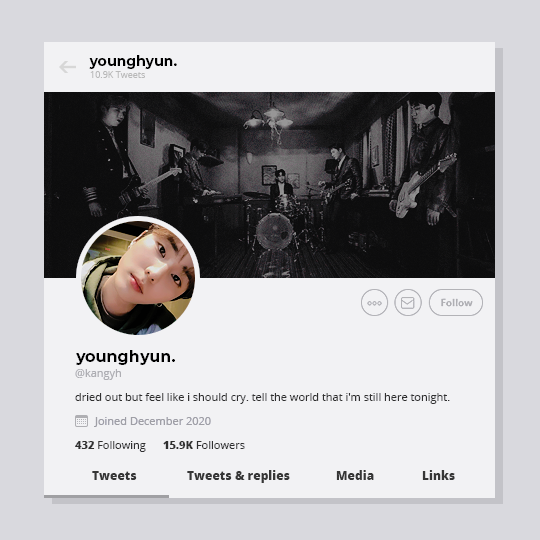The image depicts a stylized Twitter profile banner against a gray background that frames a white rectangle. The top portion of this rectangle features a gray arrow pointing to the left. Within this arrow, in black text, is the name "Young H-Y-U-N."

Beneath the arrow, "10.9K Tweets" is displayed in gray text against a backdrop of a black and white image of a band comprising four members. The drummer sits centrally, flanked by two guitarists on either side, with one additional member positioned at a keyboard.

On the left-hand side of this profile banner, a circular avatar shows an image of an Asian individual tilting their head towards the right side of the frame. The name "Young H-Y-U-N" is again printed in black near this image, accompanied by the handle "@K-A-N-G-Y-H" in gray text.

Below, a black text status reads: "Dried out, but feel like I should cry, tell the world that I'm still here tonight." Additional information in gray states: "Joined December 2020."

At the bottom of the profile, in black text, the following statistics are displayed: "432 Following" and "15.9K Followers." The footer area features several tabs labeled "Tweets," "Tweets & Replies," "Media," and "Links," along with two circles—one containing three dots, the other an envelope icon. An oval button labeled "Follow" in gray text is positioned next to these icons.